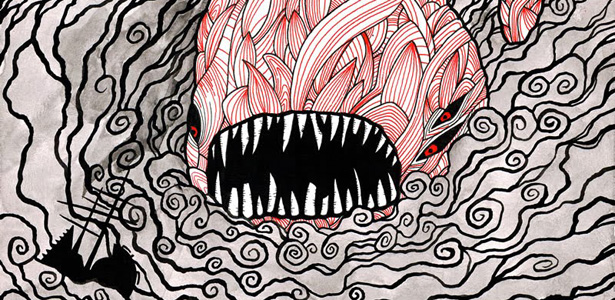This is a unique, highly detailed drawing of a fearsome sea monster, done in pen or marker with red and black ink, resembling a style influenced by traditional Japanese or Chinese art. The background is a gray hue, overlaid with swirling black lines that mimic waves or smoke. The sea monster, central to the composition, features three slit-like eyes—two on one side of its slightly turned head, and one on the other. These eyes showcase black sclera with red irises and black pupils. Its wide-open, gaping mouth is filled with two rows of sharp, jagged white teeth contrasted against the blackness inside the mouth. The body of the creature is adorned with intricate, flame-like red patterns reminiscent of scales, layered like petals or papier-mâché, extending from its fins to its tail. Breaking through the tumultuous waves, the monstrously large beast dwarfs the small, silhouetted ship in the bottom left corner, which appears partially sunken, with poles sticking out, suggesting it's either a sailboat or an island. The entire scene evokes a sense of dynamic, impending doom as the monster heads relentlessly towards the tiny vessel amidst the chaotic swirling water.